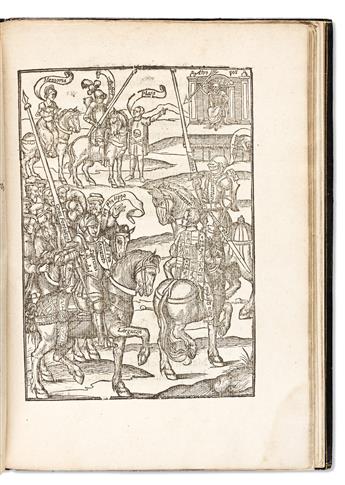The image captures a detailed scene from a medieval-themed engraving found within the aged pages of an old book. This open book, primarily showing the right-hand page, reveals intricately detailed line art. The drawing appears to depict a festive jousting event. A group of knights clad in ornate suits of armor and helmets, some raised to reveal their faces, are mounted on equally decorated horses. These knights are holding long jousting poles or lances, and they seem to be preparing for or engaged in a joust.

In the background, there's an elevated stage where a figure resembling a king sits, suggesting a place of honor or royalty. Surrounding the knights are various attendants and spectators, their heads visible as a blurred crowd. To the right, a knight on horseback, with the horse in mid-step and its head slightly forward, carries a large rod positioned vertically. In the upper section of the engraving, a small building with a man seated in front signifies additional onlookers or participants in the event. The overall scene is framed by the black trim of the open book, hinting at numerous other pages yet to be revealed. The rich, historical aesthetic of the artwork, combined with the textured, yellowed pages, evokes a strong sense of medieval pageantry and tradition.